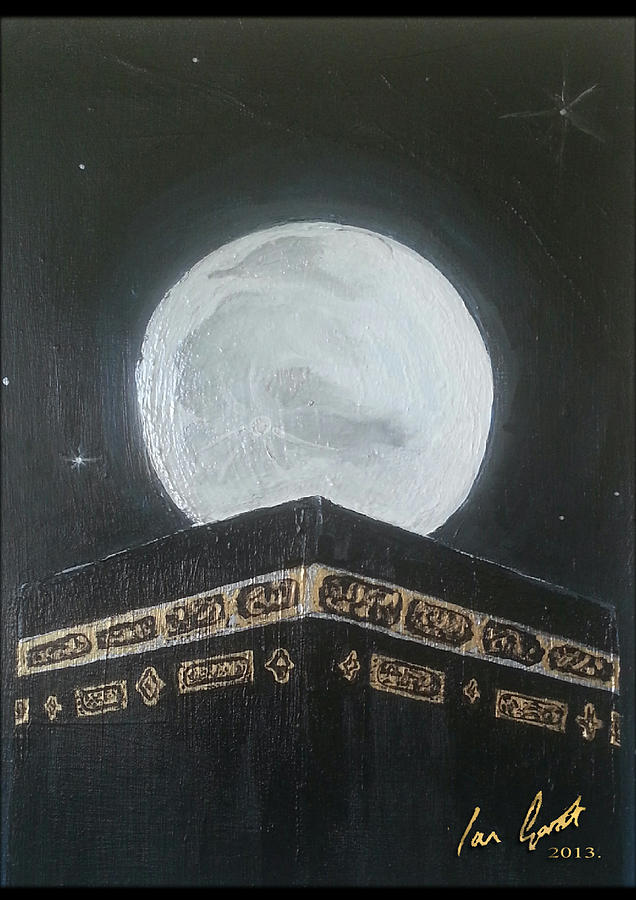This image depicts a captivating oil painting, rectangular in shape with the longer sides twice the length of the shorter sides. The artwork features a striking scene of a large moon emerging behind a box-like black tower, positioned with one of its corners directly facing the viewer. The tower is intricately adorned with two distinctive bands. The upper band consists of a solid gold strip interspersed with black ovals featuring elegant gold designs. The lower band displays an alternating pattern of gold diamonds and rectangles. Above this tower, the moon glows brilliantly, casting subtle light gray highlights over its surface. The background sky is painted in deep black, scattered with small white dots symbolizing distant stars. The painting is signed by the artist Ian Garnt in gold in the bottom right corner, dated 2013.